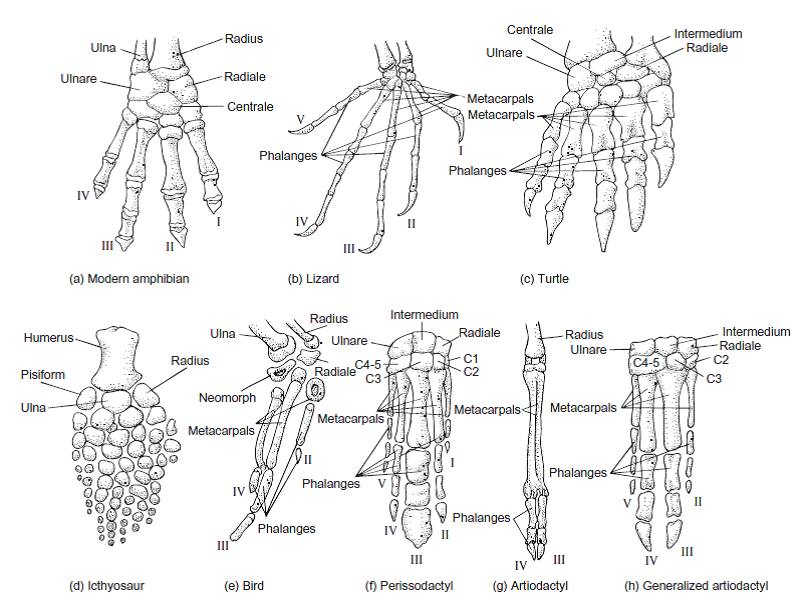This detailed illustration depicts eight different skeletons of animal feet, each labeled and exhibiting a unique bone structure. Starting from the top left, the first image shows a modern amphibian, clearly highlighting its ulna, radius, radial, ulnare, central bone, and four digits labeled with Roman numerals I through IV. Next to it, a lizard's foot is illustrated, featuring five digits labeled I through V, with detailed phalanges and metacarpals. The third image from the left is a turtle's skeletal foot, displaying its phalanges, metacarpals, ulnare, central, intermedium, and radial bones.

Moving to the bottom row, the fourth skeleton shows an ichthyosaur fin-like structure, identifying the humerus, pisiform, ulna, and radius. To its right, a bird's wing skeleton is represented, detailing the ulna, radius, neomorph, metacarpals, and phalanges. The sixth image illustrates a parasidactyl, displaying the intermedium, ulnare, metacarpals, and phalanges, suggesting a wing-like structure. Next, the artiodactyl foot is shown with its radius, metacarpals, and phalanges. Finally, the generalized artiodactyl image on the bottom right highlights the intermedium, radial, metacarpals, and lengthy phalanges. All eight skeletal structures are presented in black and white, emphasizing the intricate differences and similarities in the bone formations of these diverse animal species.